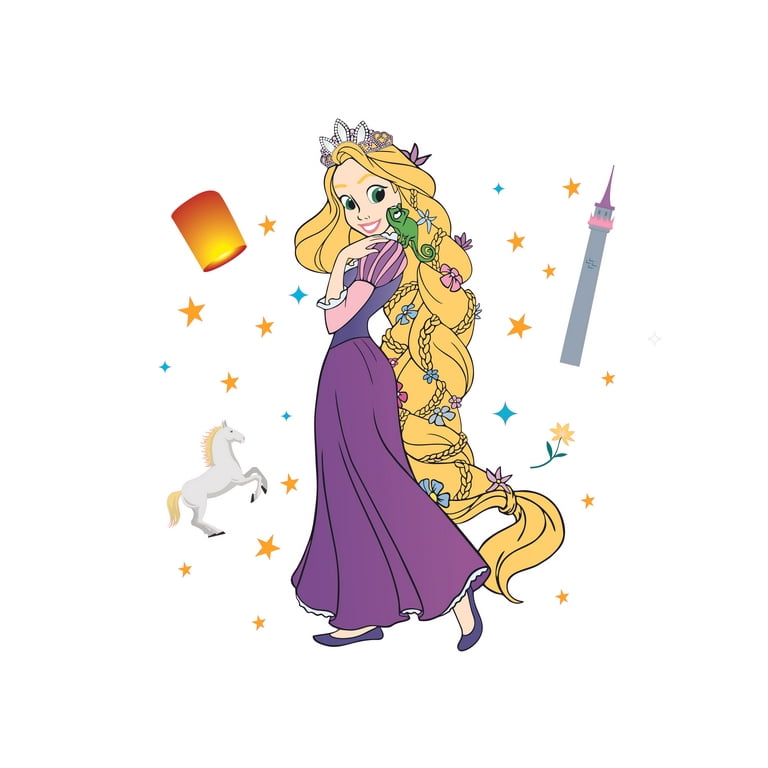The image depicts a detailed and vibrant cartoon drawing of Rapunzel, likely inspired by Disney. Rapunzel, illustrated with a white background, stands as the focal point wearing a tiara adorned in white, silver, and light purple. Her distinctive long blonde hair is braided with smaller braids interwoven and decorated with purple and light blue flowers, reaching down to her feet. She has big green eyes and blonde eyebrows, enhancing her royal appearance. Rapunzel is dressed in a purple dress with puffy purple and pink sleeves, complemented by dark purple upper portions, and matching slipper shoes. Perched on her shoulder is a small green iguana, to whom she smiles warmly, indicating a charming friendship.

The background is sprinkled with gold and a few blue stars, as well as a cheerful yellow and green flower. To her right stands a tall, whimsical cartoon tower. To her left floats an orange and yellow lantern and a small white unicorn, adding elements of magic to the scene. The overall color palette includes bright shades like black, white, blue, pink, purple, green, orange, yellow, and red, contributing to the lively and enchanting ambiance of the drawing.